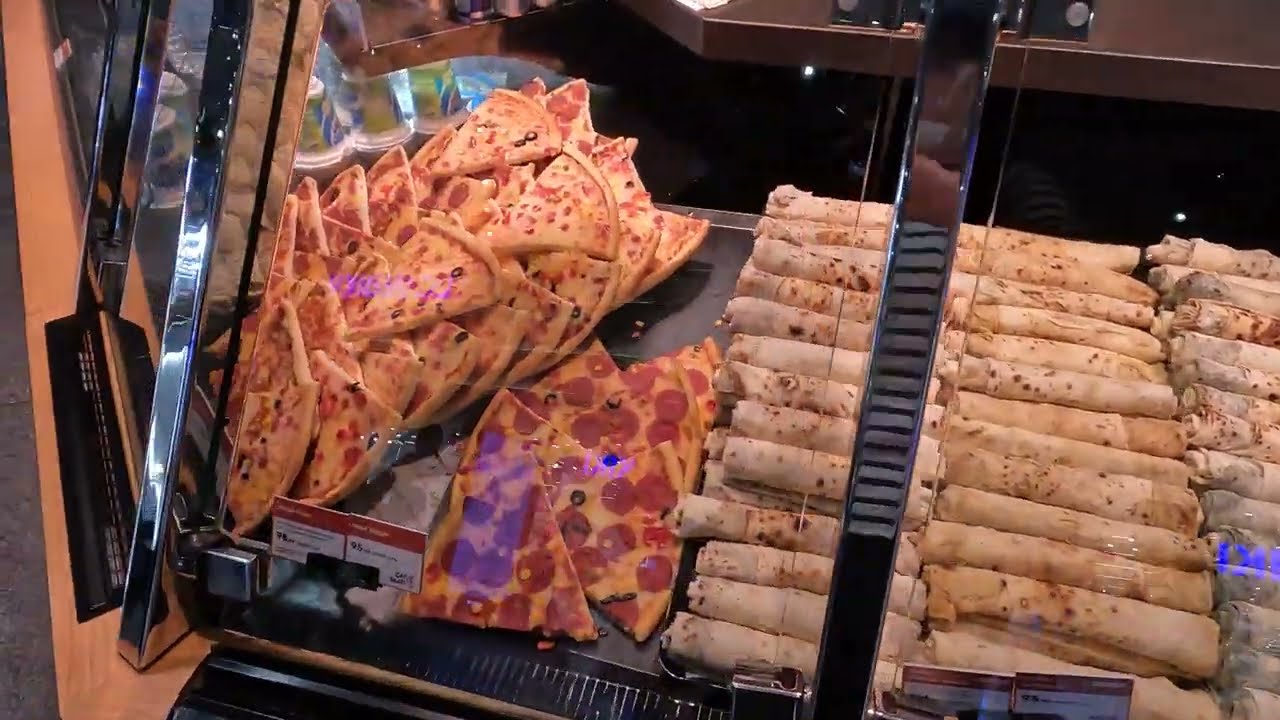This image showcases a glass display at what appears to be a deli, restaurant, or grocery store, featuring an assortment of food items. On the left side of the glass case, there are stacked slices of pizza, including both cheese and pepperoni varieties. The cheese pizza has a yellowish hue, while the pepperoni pizza is spotted with red tomato sections. To the right of the pizzas, there are rows of rolled bread items or possibly burritos, which are light in color with small brown dots, and appear to be made from a flowery dough. The glass case itself is partially open to possibly release moisture and is supported by a shiny silver metal frame. The external structure of the case features wood elements. Price tags with white, red, and black lettering describe the food items inside. Behind the display, there is a work area or table, providing a glimpse into the functional space of the stand. The ground on the left side of the image shows an orange and gray color pattern.